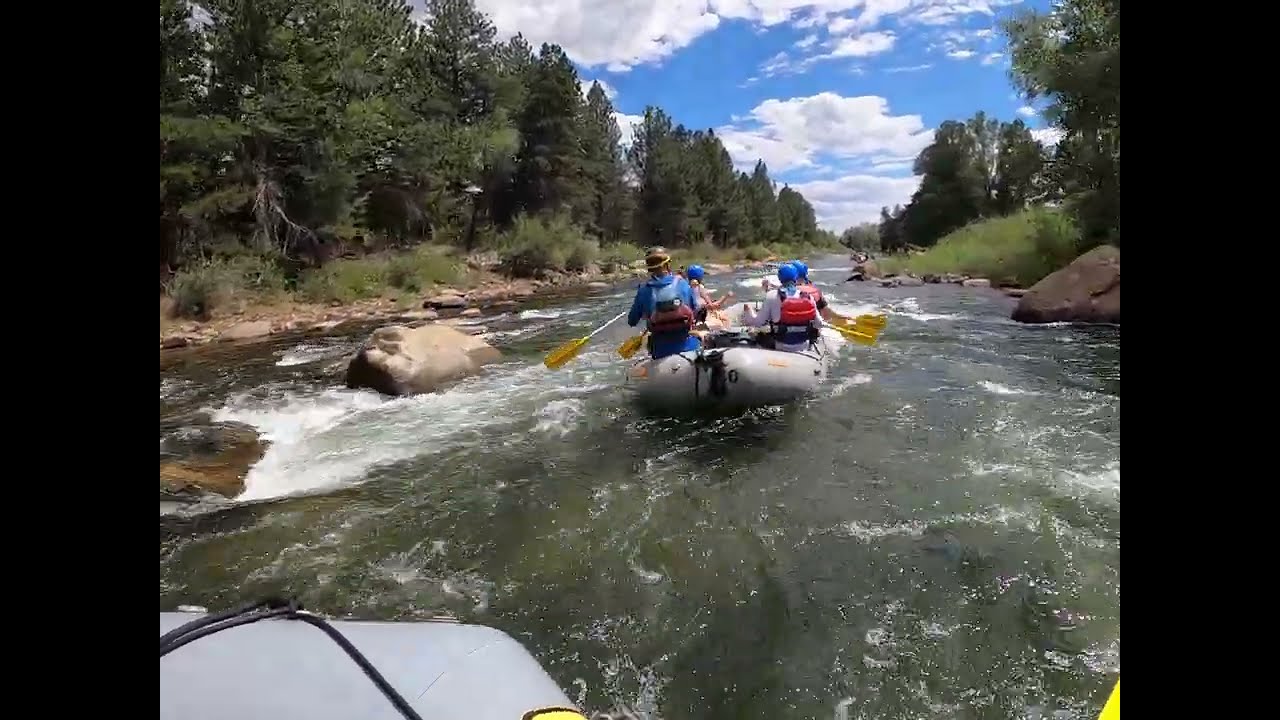In this image, a group of whitewater rafters navigates a river amidst gentle but noticeable rapids on a sunny day with intermittent clouds. The water, greenish in hue, churns around scattered rocks, creating bubbles and waves that add to the excitement. The front raft, clearly visible in the image, holds four people—likely including a guide—who are actively paddling, with those on the left side wielding their oars on the left and those on the right doing the same. Just ahead of them, another raft with four people is also visible, their paddles slicing through the water as they maneuver downstream. The scene is framed by a coniferous forest, with pine trees and tall grass lining the riverbanks, and a hint of blue sky peeking through. In the bottom left-hand corner, the front edge of another raft can be seen, along with a rafter holding a camera, presumably capturing the thrilling adventure. The overall atmosphere suggests a fun and exhilarating outdoor experience in a picturesque natural setting.